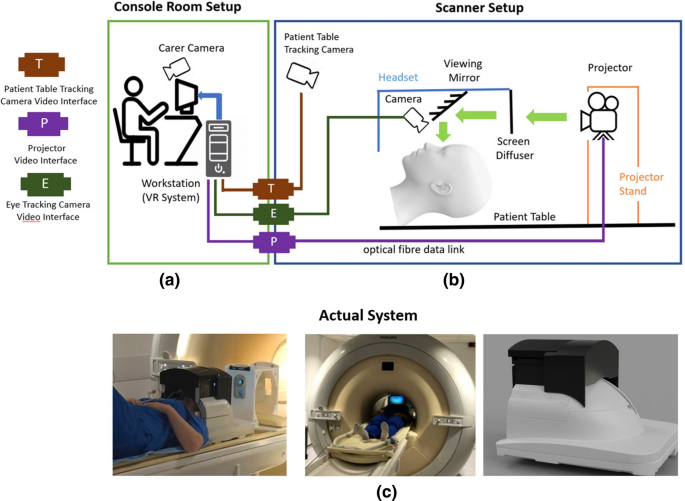The image is a composite that illustrates the setup for a likely CAT scan facility designed for head studies, emphasizing both the detailed diagram at the top and the actual system overview at the bottom. In the top section, the stylized diagram features interconnections of the equipment. On the left, an operator sits at a computer workstation labeled "workstation (VR system)," being monitored by a "carer camera." Three lines extend from the computer to a wall pass-through, marked as "T," "E," and a purple line. "T" connects to the "patient table tracking camera," while "E" links to an "eye tracking camera" within the headset area, which also contains a diagonally placed mirror. The purple line leads to a projector that displays images through green arrows, reflected onto the patient’s eyes via the viewing mirror. 

Below this, the image is labeled "actual system," depicting three photographs: 
1. A patient in a blue outfit lying on a table with a head structure.
2. The same patient being moved into the circular ring of the scanner, possibly a CAT scan or MRI.
3. A close-up of the head structure, showing a white plastic cover with a black top that houses the camera and viewing mirror. 

Additional details include the workstation setup, VR system, projector, screen diffuser, and an optical fiber data link, all connected and color-coded in blue, green, and pink line drawings against a white background.